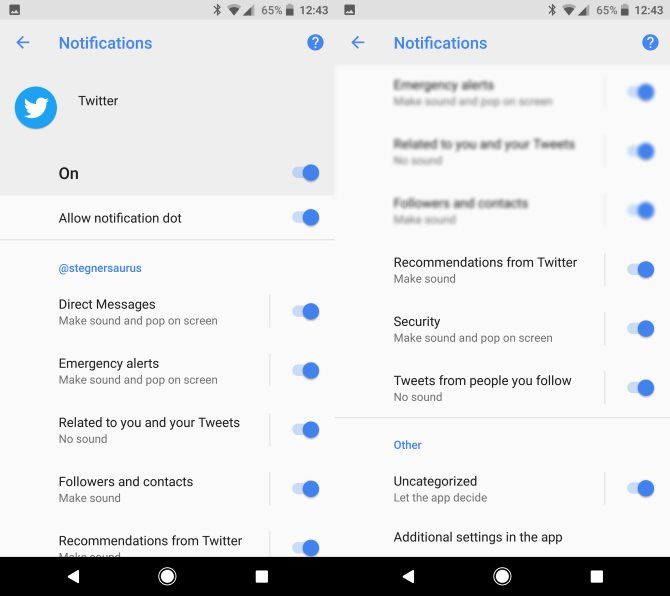Two side-by-side screenshots display identical system notifications at the top, including a Bluetooth symbol, Wi-Fi icon, battery level at 65%, and the time "12:43". Both images have a gray and white background with blue and black text elements.

On the left screenshot, the top section starts with a blue arrow pointing to the notifications. This is followed by a blue circle with a white question mark, and a blue circle featuring a white bird icon next to the word "Twitter". Below these icons, a list of notification settings is shown, each highlighted with a blue circle:
1. "On" – Allows notifications.
2. "Allow notification dot" – Marked for "@STEGNERSAURUS" in blue.
3. "Direct messages" – Makes sound and pops on screen.
4. "Emergency alerts" – Makes sound and pops on screen.
5. "Related to you and your tweets" – No sound.
6. "Followers and contacts" – Makes sound.
7. "Recommendations from Twitter" – Makes sound.

Both images feature a black bar at the bottom, spanning across them, containing three white icons: a triangle, a circle, and a square.

The right screenshot presents the same notification indicators and icons as described earlier. However, the first three menu items are grayed out and slightly blurred:
1. "Emergency alerts"
2. "Related to you and your tweets"
3. "Followers and contacts"

Further down, the following options appear clear and distinct, with blue circles beside them:
4. "Recommendations from Twitter" – Makes sound.
5. "Security" – Makes sound.
6. "Tweets from people you follow" – No sound.
7. "Other" – Marked in blue.
8. "Uncategorized" – Allows the app to decide.

Finally, it mentions "Additional settings in the app" at the bottom.